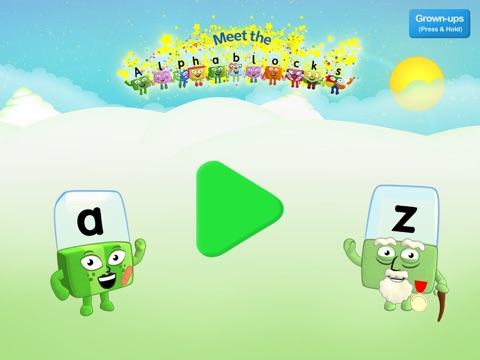Screenshot from a webpage depicting a colorful and engaging scene from "Meet the Alpha Blocks." In the upper right-hand corner, a prominent blue button labeled "Grown-ups" in white text is accompanied by a smaller instruction in parentheses that reads "(press and hold)." The top of the page features the title "Meet the Alpha Blocks" adorned with bright yellow glitter.

Beneath the title, a cast of vibrantly colored characters known as Alpha Blocks is displayed. Each character is uniquely colored and designed with a squarish head, featuring eyes, a mouth, arms, and legs, effectively exhibiting their playful and animated nature.

In the background, a sun peeks from the upper right corner above a sky dotted with white clouds. The lower section of the background transitions from a light green to a very light white, suggesting a grassy hill.

Prominently positioned are two specific Alpha Blocks: On the left, a green block with dark and light green stripes stands out. This character has two arms and legs, black eyes with white irises, a mouth, and a lowercase "a" enclosed in a clear box above its head. On the right, another figure shares the same block-based design but with older features—white eyebrows, lines under its eyes, a nose, and a white beard. This character is holding a cane and has a lowercase "c" in a clear box above its head.

In the middle of the scene, a large green triangle points to the right, adding a dynamic element to the composition.